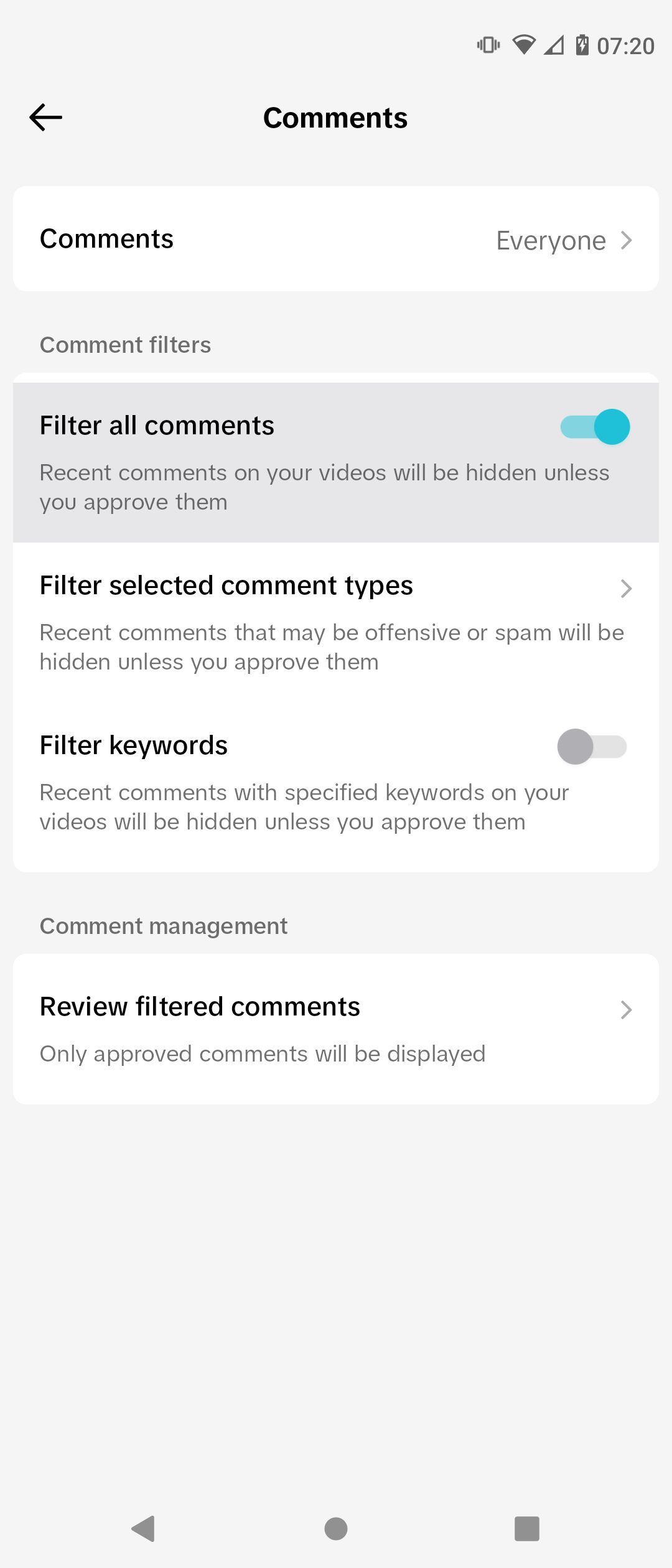This image is a screenshot from a mobile device depicting the "Comments Settings" menu. 

At the top right corner, the screen displays a light gray bar indicating a resolution of 720p. The battery icon shows it is nearly full and currently charging. The Wi-Fi signal, represented by three bars, and the Internet connection, indicated by one bar, are visible. The phone is set to vibrate mode. 

On the left side of the screen, there is a back arrow pointing to the left. Centrally, the word "Comments" is displayed in bold black text. Below it, a white bar spans the screen, with "Comments" written in black on the left, and "Everyone" with a greater-than symbol on the right, indicating a drop-down menu.

The background of the next section is light blue. On the left, in black text, it reads "Comment Filters." Below is a thin white bar, followed by a light gray area. In bold black text, it states "Filter All Comments," with the toggle switch activated and highlighted in light blue. 

Underneath, it reads "Recent comments on your videos will be hidden unless you approve them" in regular black text. There is a white rectangle beneath this, with "Filter Selected Comments" in bold black text at the top left and a greater-than symbol on the right side. Below this heading, two lines of gray text provide additional details.

Further down, “Filtered Keywords” is boldly printed in black text, with the toggle switch turned off. Underneath, two gray lines describe further information. 

The next section is labeled "Comment Management" in black text on a blue background. An adjacent white rectangle says "Review Filtered Comments" in bold, with a greater-than symbol on the right side. Below, it notes "Only provided comments will be displayed" in small black text.

Finally, at the bottom of the screen, there are three inches of light blue background. A gray circle, a left-pointing gray triangle, and a gray square are aligned towards the bottom.